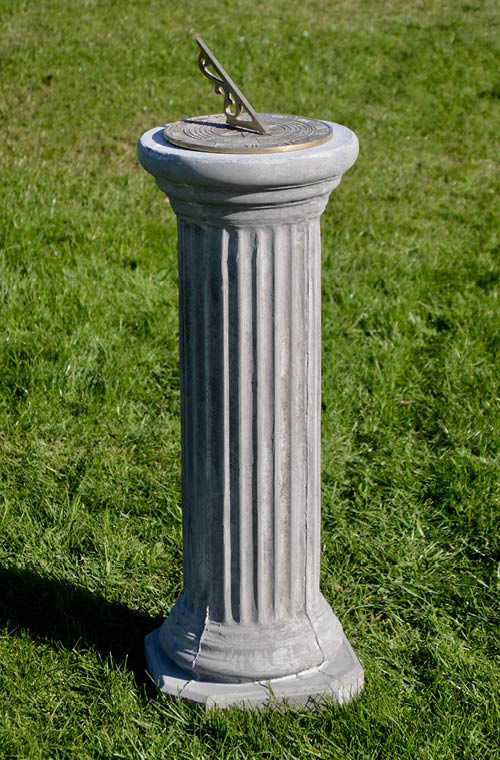The image depicts a historical sundial set atop an ornate, waist-high pedestal reminiscent of ancient Roman or Greek architecture. The pedestal, likely made of concrete or stone, features ingrained indentations and stands prominently in the middle of a vast, green field with some patches of brown grass scattered in the background. The gray-colored sundial, with its intricately designed metal gnomon, casts a clear shadow indicating the time, likely around noon. The scene is illuminated by abundant sunlight, further emphasizing the shadow cast by the pedestal on the well-maintained, short grass surrounding it. The open field lacks any trees, offering an unobstructed view ideal for the sundial's function of tracking the sun's movement.